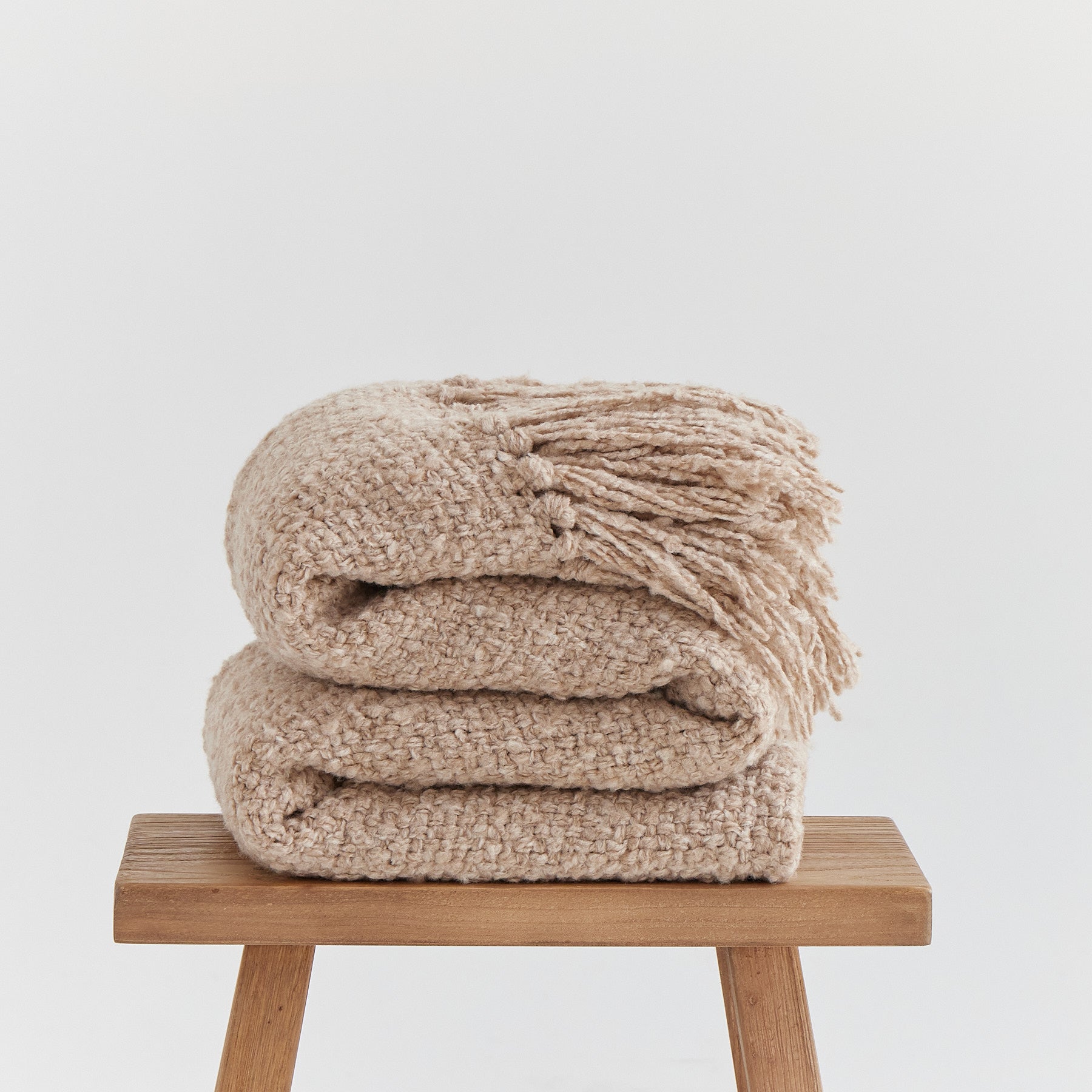In the image, a small, simple wooden bench with a curved seat and two supporting legs stands against a light gray background, evoking the atmosphere of a minimalist studio setting. The bench’s surface, characterized by its horizontal wood grain, reveals a rustic charm, possibly showing subtle cracks or natural lines in the wood. Atop this bench, a meticulously folded tan afghan, tinged with hints of whitish-gray, is prominently displayed. The afghan, resembling a handwoven creation, boasts long, knotted tassels approximately six inches in length along its edge, adding a touch of intricate detail. The blanket occupies most of the bench, emphasizing the bench’s compact size. This carefully staged scene, devoid of any text or human elements, appears designed for a sales catalog or advertising, highlighting both the rustic bench and the cozy, textured afghan as the central subjects.